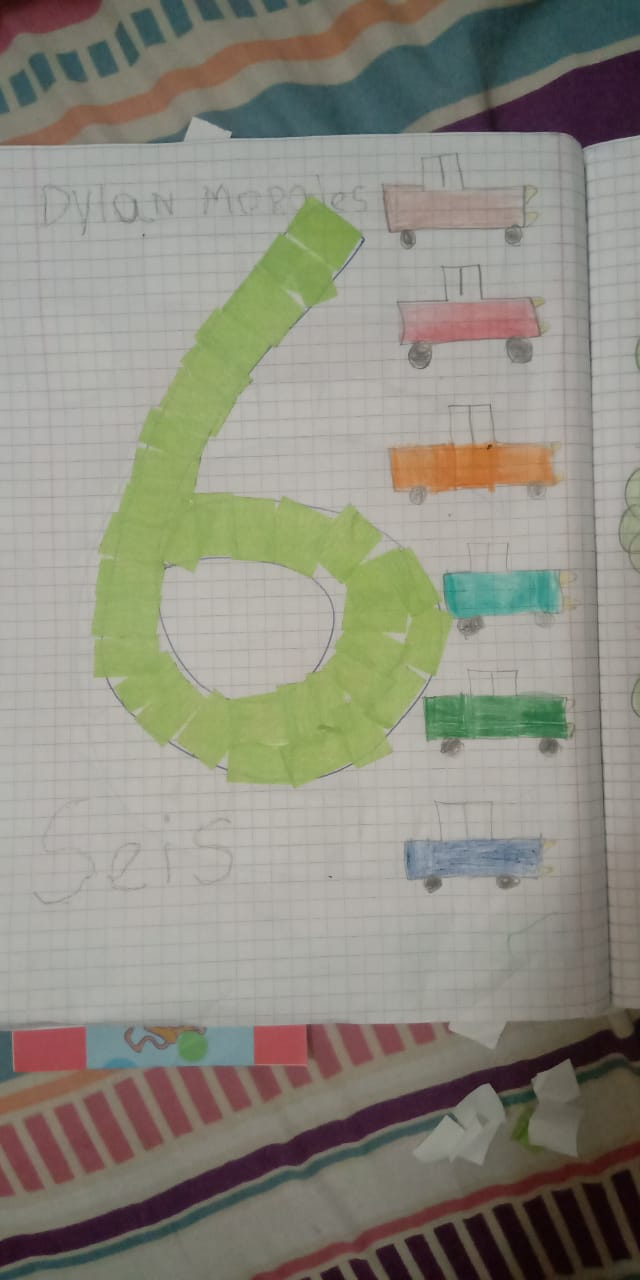This image shows a page from a graph paper notebook that is bound, possibly spiral-bound, resting on a tablecloth. The tablecloth features a pattern of vertical bars and horizontal stripes in dusty blue, peach, and burgundy. At the top of the page, "Dylan Morales" is written in pencil. The focal point of the page is a large, irregularly shaped number six outlined in pen. The interior of the six appears to be filled with small pieces of tape, possibly green paper. Along the right-hand side of the number, Dylan has drawn six boxy cars or trucks, neatly arranged in a vertical column. These vehicles are various colors: pink, red, orange, turquoise, green, and dark blue. In the bottom left-hand corner, the word "Faith" is penciled in. The tablecloth’s design complements the child-like drawings and text, providing a colorful backdrop with its white, maroon, pink, and blue segmented patterns.